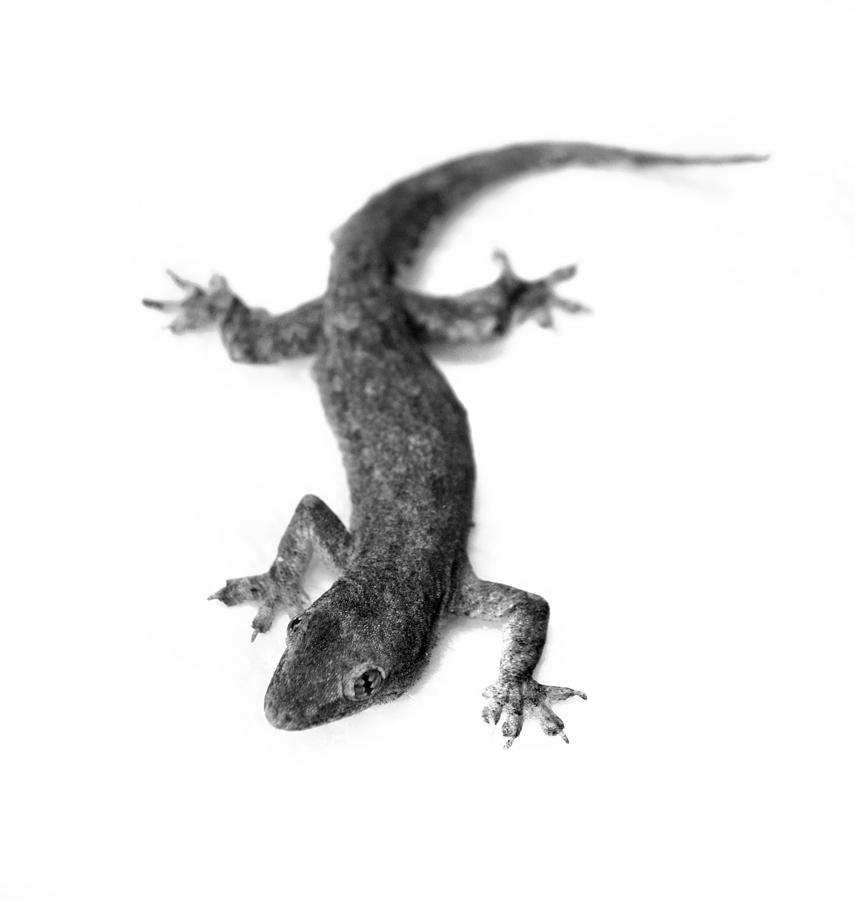The black-and-white image features a lizard, most likely a gecko or possibly a salamander, in a nuanced grayscale palette. The lizard's body exhibits different shades of gray, with some patches appearing darker than others. Its vertically slit pupils, pronounced and bumpy, add significant detail to the creature's gaze, suggesting possible false eyelids around them. The lizard's head is pointed towards the lower left of the frame, giving the impression of facing the viewer slightly to the left, while its elongated body curves, leading to a tail directed towards the upper right of the picture. The clarity of the image varies, with the head being sharply focused and the midsection to the tail appearing blurry. The lizard's limbs are distinct, with five toes on each foot, each equipped with sharp claws, visible on both the front and the back legs. The background is plain white, highlighting the lizard's form.